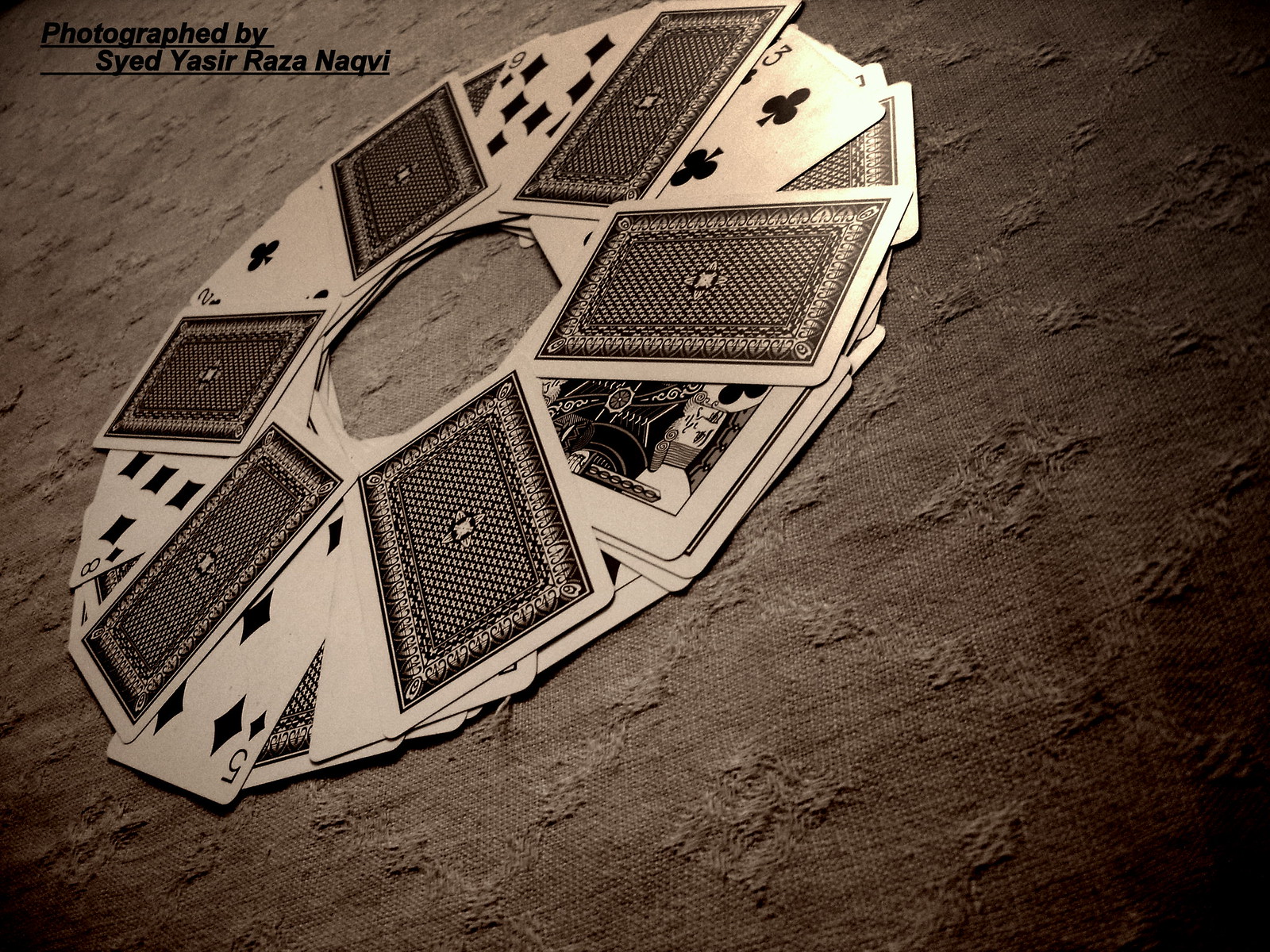In this black and white photograph by Syed Yasir Raza Naqvi, a meticulously arranged deck of playing cards is displayed on a textured tablecloth with a diamond pattern. The tablecloth features a dark gray hue and a raised threading that enhances its intricate design. The deck is laid out in a circular, alternating pattern: five cards face down, followed by six cards face up, and then another five cards face down. The backs of the cards are adorned with a detailed diamond and cross pattern, reminiscent of a finely crafted mosaic area rug. Visible cards in the arrangement include the Two of Clubs, Nine of Diamonds, Three of Clubs, King of Clubs, Five of Diamonds, and Eight of Diamonds. The distinctiveness of each card adds to the visual appeal and complexity of the composition. Notably, the corner of the image features a black underlined caption, "Photographed by Syed Yasir Raza Naqvi," crediting the artist with clear, bold typography.